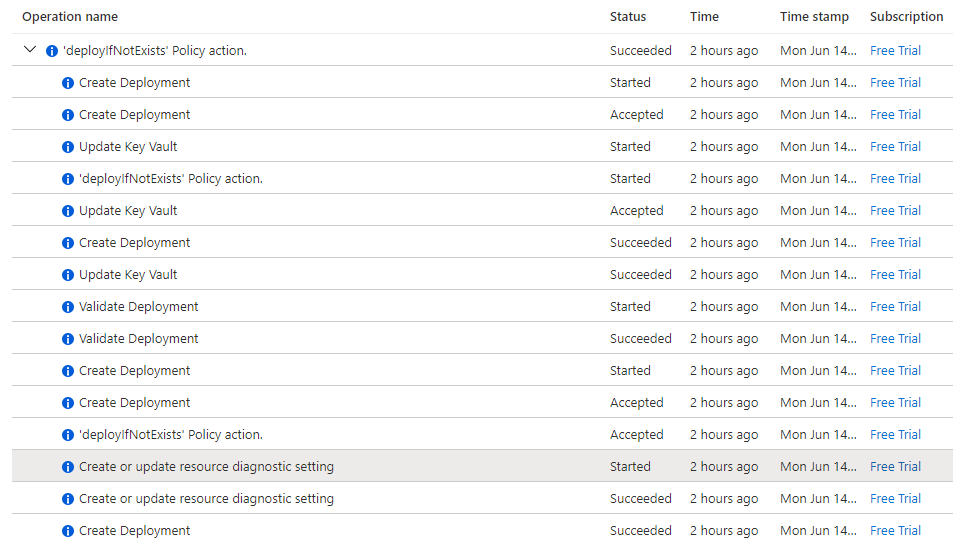**Deployment Operations Log for Project Topaz**

*Operation Name:*
- Project Topaz

*Details:*
- **Status and Title:** 
  - Various deployment and update actions as part of the trial.

*Timeline:*
- **Two Hours Ago on Monday, June 14th:**
  - **Create Deployment:** Started
  - **Get Deployments:** Accepted
  - **Update Keyfile:**
    - Starting
    - Accepted
  - **Deploy if Non-Existent Policy Action:** 
    - Started
    - Succeeded
  - **Create Deployment:** Succeeded
  - **Validate Deployment:** Started
  - **Create or Update Resource Diagnostic Setting:**
    - Started
    - Created/Updated succesfully

*Subscription:*
- Details of the policies and deployments linked to the subscribed service.

*Log Summary:*
- There is a text table showing the deployment status and operations with *16 rows* and *5 columns*. The following operations are logged sequentially in the table for better overview and tracking purposes:

1. Create Deployment
2. Get Deployments
3. Update Keyfile (Starting)
4. Update Keyfile (Accepted)
5. Deploy if Non-Existent Policy Action (Started)
6. Deploy if Non-Existent Policy Action (Succeeded)
7. Create Development (Succeeded)
8. Validate Deployment (Started)
9. Create or Update Resource Diagnostic Setting (Started/Completed)

This detailed log is reflective of various deployment processes undertaken under project Topaz, ensuring all actions are successfully recorded and tracked.